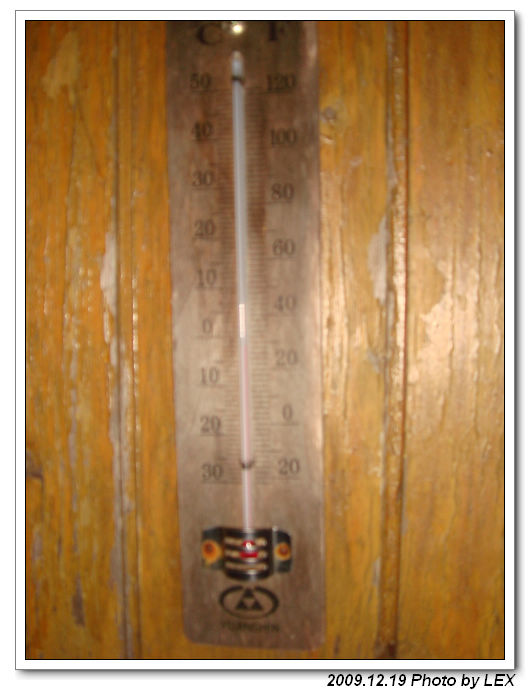In this image, we observe a wooden wall that spans the entire visual field. The wall has a light brown hue and appears to be in a state of disrepair, with noticeable tears and exposed inner sections on both the left and right sides. Centrally positioned from top to bottom is a thermometer. The background of the thermometer features a dark brown color. 

At the bottom of the thermometer, there is a black triforce symbol comprised of three interconnected triangles, enclosed within a circle. Beneath this symbol, there is an indistinct seven-letter word due to blurriness. 

The thermometer itself consists of a central glass tube with a red liquid line rising through its lower half. Numerical markings flank the thermometer: on the left side, the numbers ascend from -30 to 50 in increments of 10, while on the bottom right, the scale ranges from -20 to 120 in increments of 20. Positioned at the top left of the thermometer is the letter "C," and at the top right, the letter "F" can be seen, indicating Celsius and Fahrenheit measurements respectively.